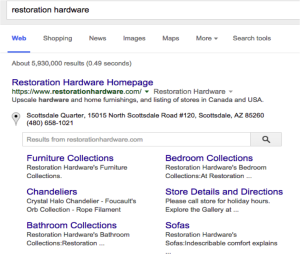Detailed Caption: 

The search result for "Restoration Hardware" prominently displays the company's official website link as the first result, identified as "Restoration Hardware Homepage." The summary includes navigation links embedded within the result, such as "Furniture Collections," "Chandeliers," "Bathroom Collections," "Store Details and Directions," and "Sofas." Additionally, the address for the Scottsdale Quarter location in Scottsdale, Arizona, along with a 480 area code phone number, is provided. The search interface features a typical white background, with blue hyperlinks, black text, and an array of search options at the top, including shopping, news, images, and webpages.